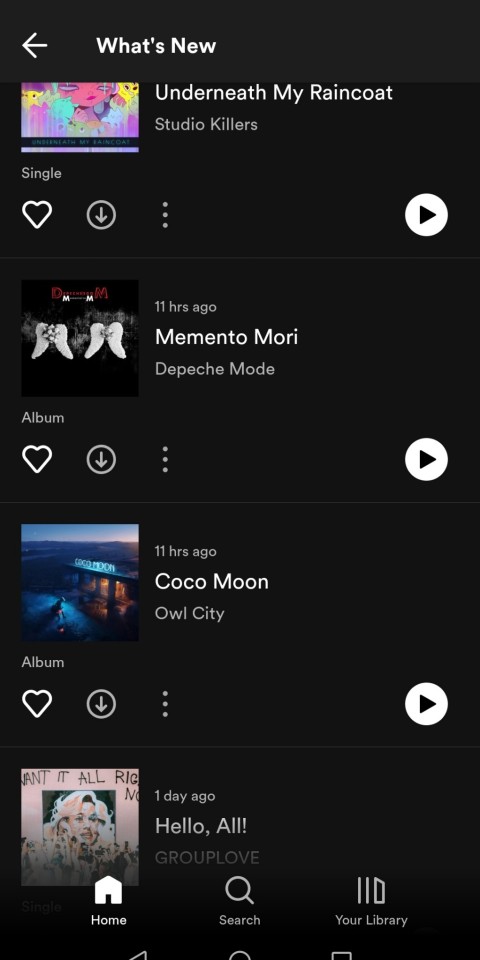This image showcases a music library interface displayed in dark mode, characterized by an all-black background. 

At the top of the screen is a navigation arrow pointing to the left, facilitating a return to the previous page. Adjacent to the arrow is the text "What's New," indicating the section's purpose. 

Beneath are four distinct cards, each representing a different song. Each card includes an image of the cover art related to the respective song. Below the cover art, details such as the song's title, the artist's name, and possibly the last played time are displayed.

Each song card also features several interactive icons: a white outlined heart for favoriting the song, a download icon for offline access, and a vertical ellipsis (three dots) for additional options. To the right is a solid white play button with a black triangle in the center, allowing immediate playback of the song.